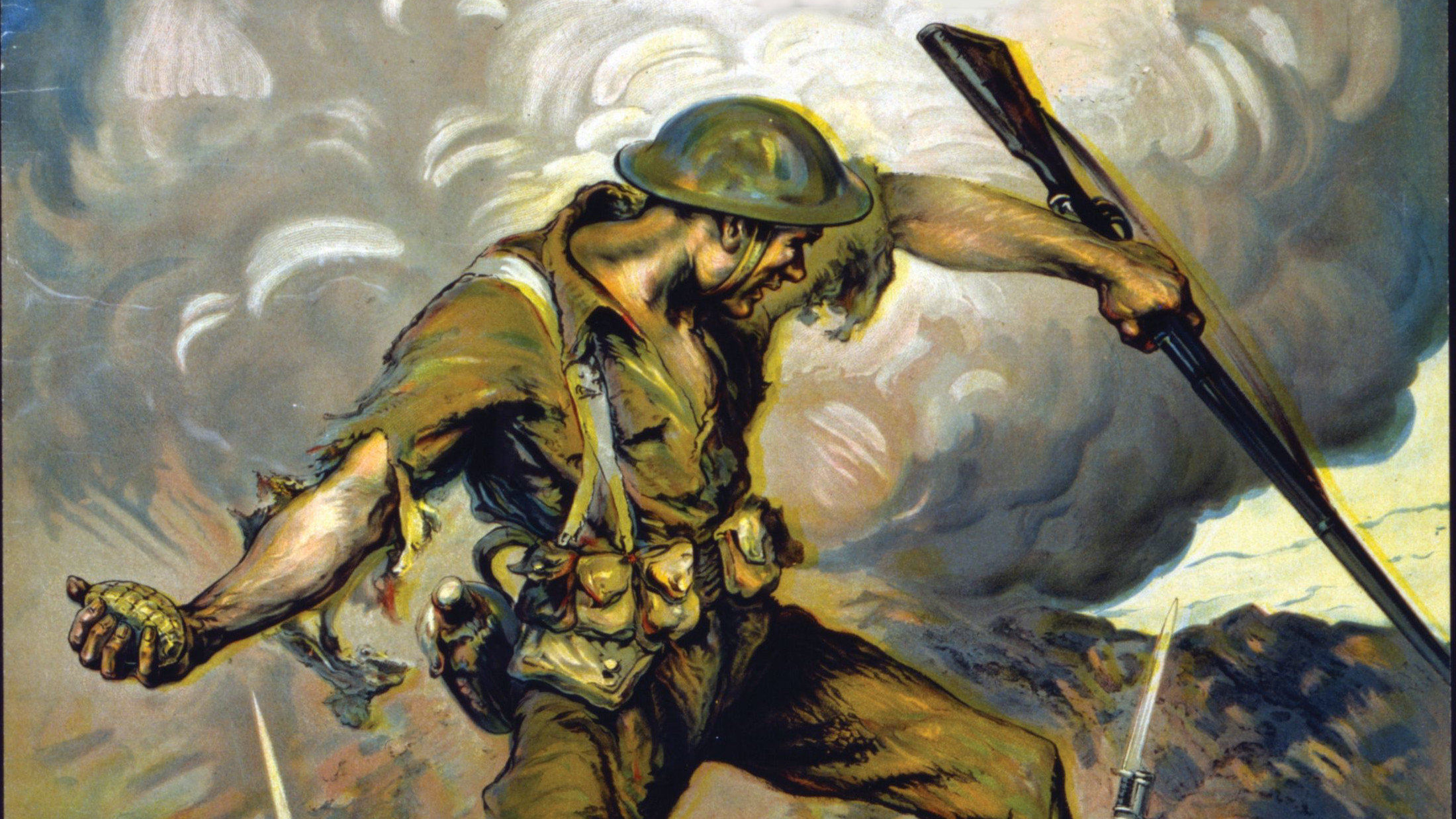This detailed watercolor painting portrays a soldier from an older era, likely from the 1930s or earlier, wearing a tattered and torn uniform. His olive, forest green shirt is shredded at the elbows, and he wears a helmet reminiscent of the World War I era. The soldier's belt, supported by suspenders, is loaded with various attachments, including a canteen. In one hand, he clutches an M1 Garand rifle, while the other is poised to throw a grenade. Surrounding him, the tips of rifles with bayonets are visible, underscoring the tension of the scene. A massive, black plume of smoke from an explosion billows in the background, adding to the chaotic atmosphere.